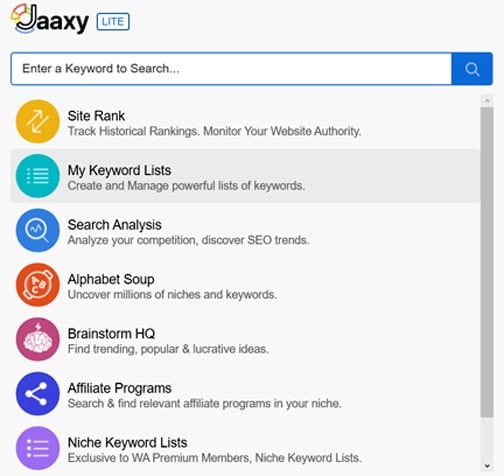In the upper left corner of the image, a large letter "J" is situated, followed by the letters "A-A-X-Y" next to a blue square that spells out "L-I-T-E." The background is predominantly white, accentuating the black text that prompts users to "enter a keyword to search." Accompanied by a blue square and the phrase "mental angular," this section establishes the context for a search functionality.

The top left also features a graphical element in yellow consisting of an arrow that points upward, rightward, and downward. Adjacent to this, text advises users to "track historical rankings" and to "monitor your website authority." 

Moving further, a blue circle with repetitive text that appears as "jah, jah, jah" suggests a bio-keyword list, guiding users to "create and manage powerful lists of keywords." This is followed by a blue circle containing a magnifying glass icon and a dash bar representing a search analysis tool. The text here encourages users to "analyze your competition" and "discover SEO trends." 

A red circle contains the phrase "alphabet soup" within it, indicating a feature designed to "uncover millions of niches and keywords." 

To the right of this, a purple circle encloses a brain icon, labeled as "Brainstorm HQ," which assists users in finding trending, popular, and emerging ideas. 

The background features a blue section highlighting "affiliate programs," where users can "search and find relevant affiliate programs in your niche." Another purple circle adorned with "jah, jah, jah" text points towards an exclusive offer labeled "NicheKeywordList," which is specifically available to Washington premium members. This section concludes with a gray bar. 

Overall, the image provides a comprehensive set of tools and features focused on keyword management, SEO analysis, and affiliate program discovery, all visually organized with distinctive colored circles and informative text.